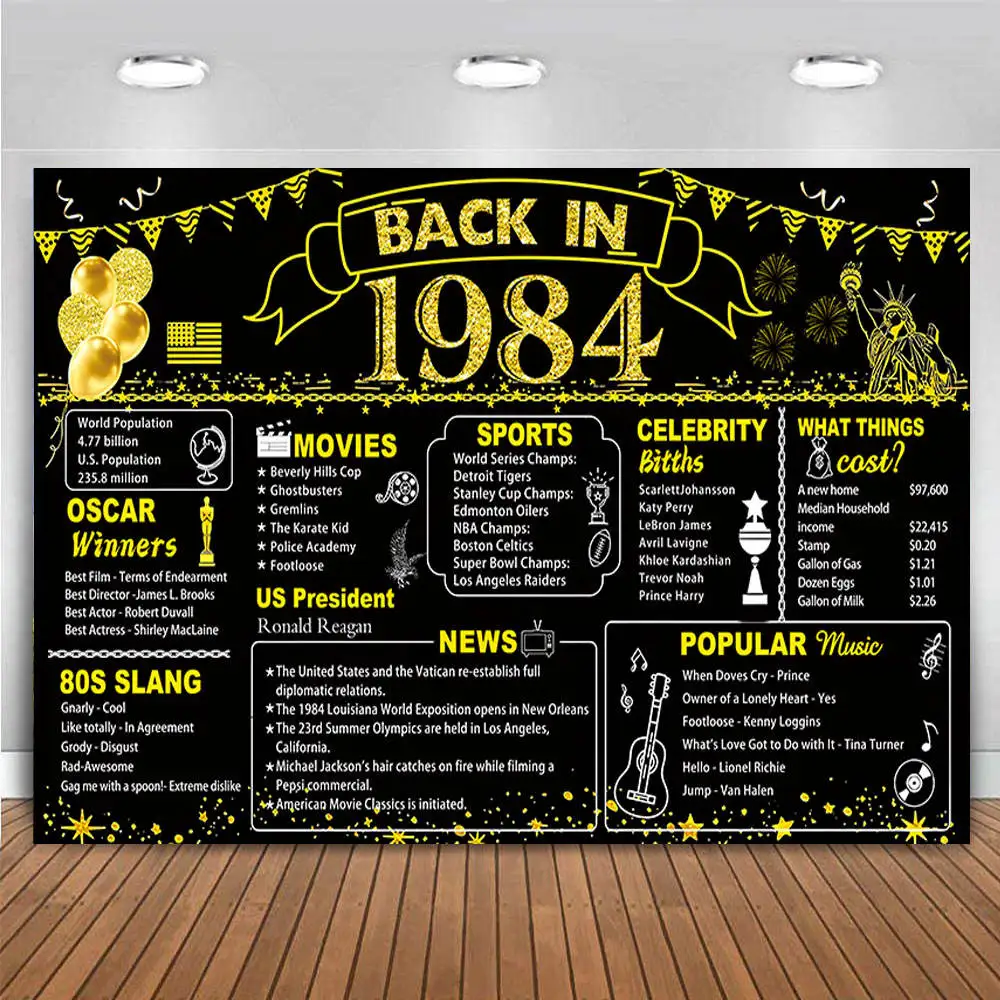This vibrant color photograph features an intricate display set against a greyish wall adorned with three rectangular, silvery elements that may be lights. Below these elements lies a spacious wooden floor.

Dominating the scene is a large, eye-catching sign with a black background and accented by white and yellow text. At the center top of the sign, the phrase "Back in 1984" is prominently displayed. The upper left corner is decorated with a cluster of yellow balloons, and festive bunting stretches across the top edge, adding a celebratory touch.

The sign is divided into several sections, each detailing notable events and trivia from the year 1984. Key sections include:

- **Oscar Winners**: The header is in yellow, with specific award recipients listed in white text beneath it.
- **80s Slang**: Highlighting popular phrases of the decade.
- **Movies**: A list of notable films from the year.
- **US President Ronald Reagan**: Featuring information about the sitting president.
- **News**: Enclosed in a boxed section towards the bottom middle-right.
- **Sports**: Summarizing key sports events.
- **Celebrity Births**: Recognizing famous individuals born in 1984.
- **What Things Cost**: Providing a glimpse into the prices of various items during the year.
- **Popular Music**: Including tracks like "When Doves Cry" by Prince and "Footloose" by Kenny Loggins. This section is adorned with a small picture of a guitar.

Each section is enhanced with small illustrations corresponding to its theme, such as award statues and sports balls, contributing to the engaging and nostalgic nature of the display.